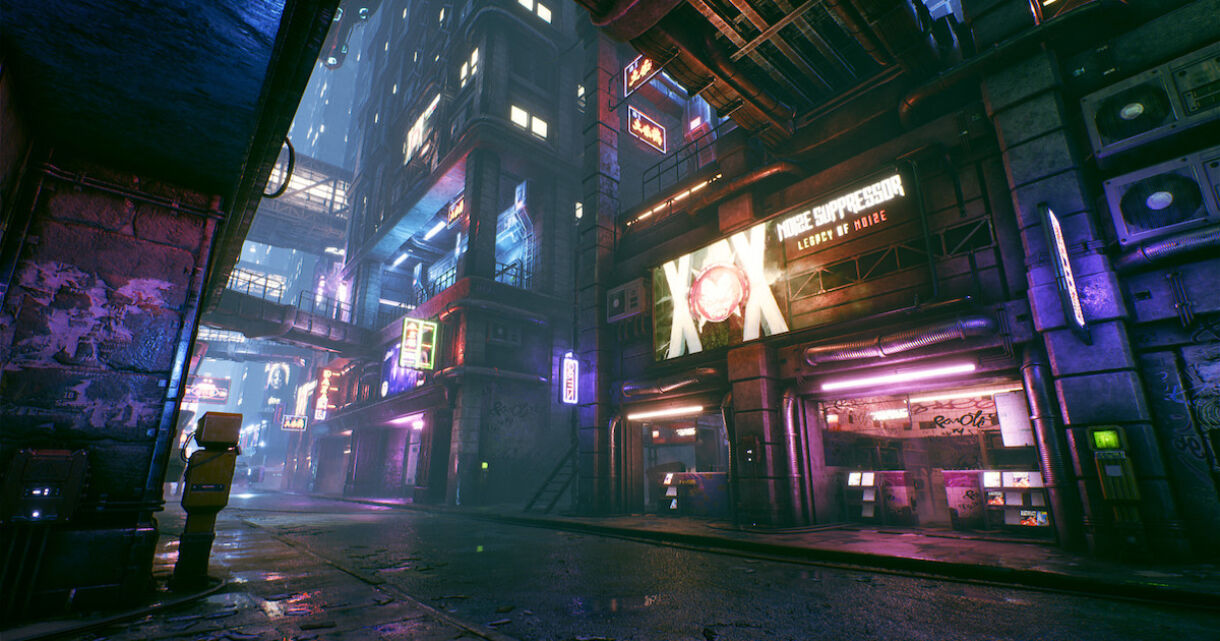This image depicts a futuristic, dystopian urban scene at night, likely inspired by a city in Japan. The streets are filled with a palette of dark blues and purples, illuminated by vibrant neon lights. Prominently displayed is a sign with white, digital-looking X's, although the full message is unreadable due to the glow. A tall, rectangular skyscraper reaches into the sky next to this sign. The cityscape is interconnected by skywalks and pedestrian bridges, some open-air and others fully enclosed, bridging the gaps between towering buildings. On the ground level, the cement street and visible sidewalk are lined with various lit-up shops, including one with the partially discernible banner "XOX" and another small shop with pink chairs inside. A stark stone wall appears on the left, adding texture to the scene, while a robot stands sentinel on a corner, enhancing the futuristic ambiance. The overall atmosphere is dark and dystopian, with the glow from LED lights providing the only respite from the shadowy surroundings.